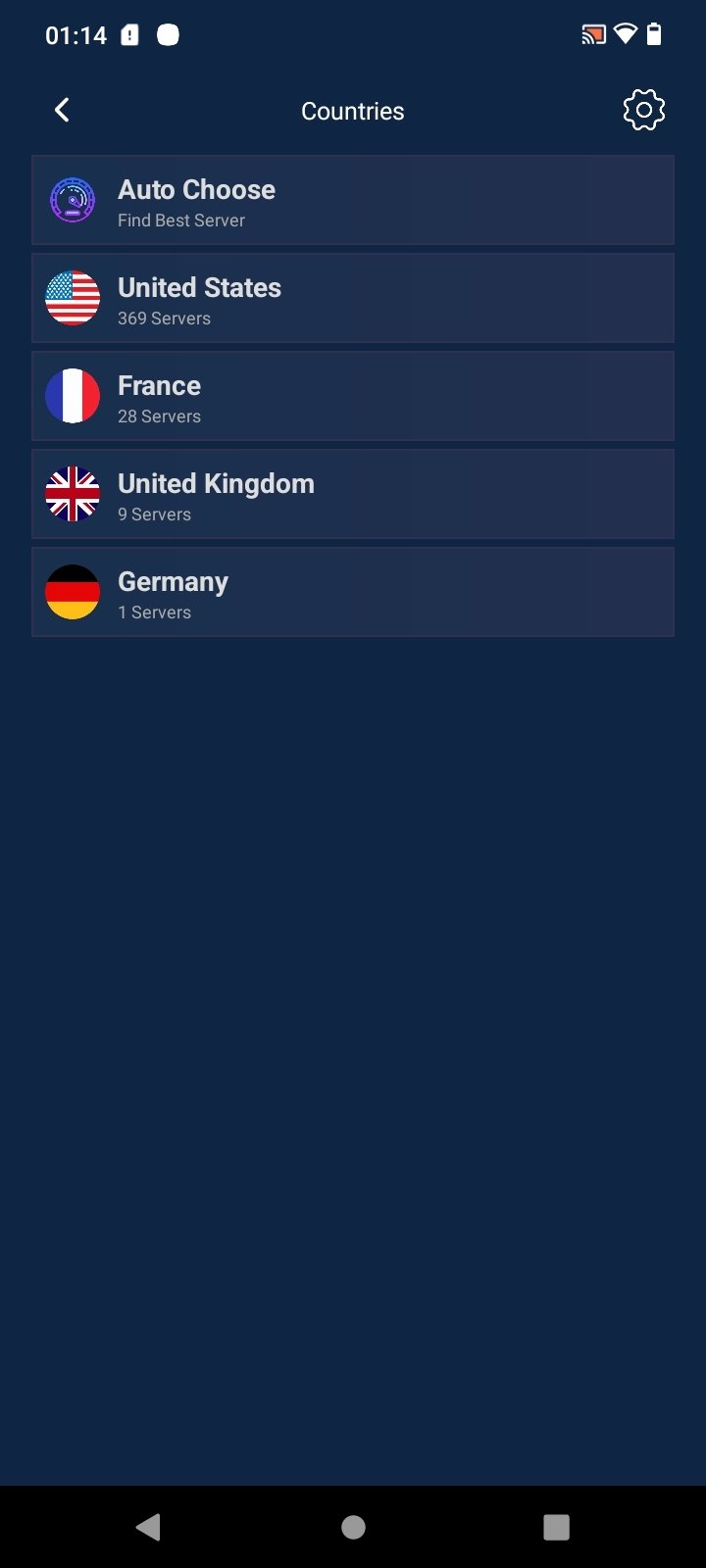The image features a dark blue background. In the top left corner, there is a digital clock displaying "01:14" alongside two unidentifiable icons. On the upper right side, there is a gray and orange icon. The Wi-Fi signal icon, near-full but not completely, is visible next to an almost full battery icon.

Centered beneath these icons is a less-than symbol ("<"), followed by the word 'countries' positioned in the middle of the screen with a settings gear icon just to its right. Below this is a gray box containing the text "Auto choose find best server," with a purple round icon to its left.

Further down the screen, the image lists various countries along with their respective flags and the number of servers available:
- The United States flag with "United States" and "369 servers"
- The French flag with "France" and "28 servers"
- The United Kingdom flag with "United Kingdom" and "9 servers"
- The German flag with "Germany" and "1 server."

The rest of the image is empty space.